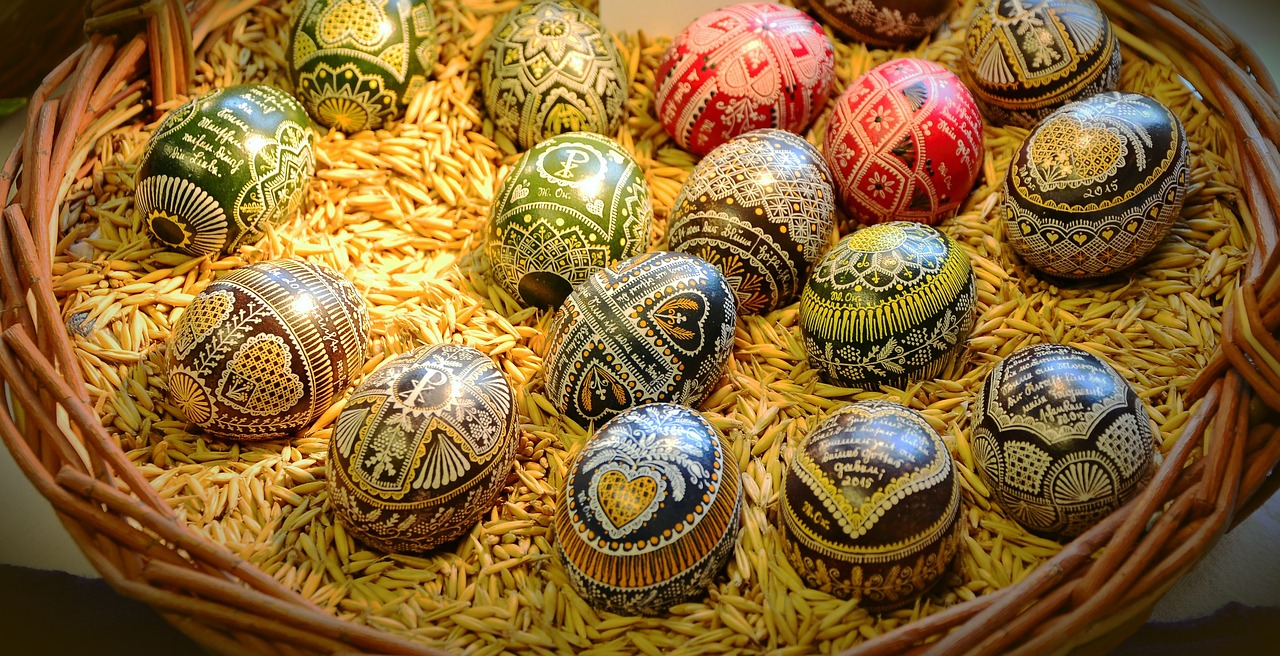This photograph captures a beautifully woven, reddish-brown wicker basket filled with yellowish-beige grains or pieces of orzo, cradling an assortment of intricately decorated eggs. The eggs, positioned artistically within the basket, showcase elaborate white and gold patterns against vibrant jewel-toned backgrounds. Dominating the arrangement are five black eggs forming an arc at the bottom, and another cluster of five black eggs near the top right. The top left holds four emerald green eggs, while the center top features two striking ruby red eggs. Notably, one egg is inscribed with the year "2015" in elegant white text. The overall design of the eggs exudes a mix of Pennsylvania Dutch and Russian folk art styles, with a homey, cozy vibe, each egg meticulously painted and brimming with cultural and possibly biblical themes.